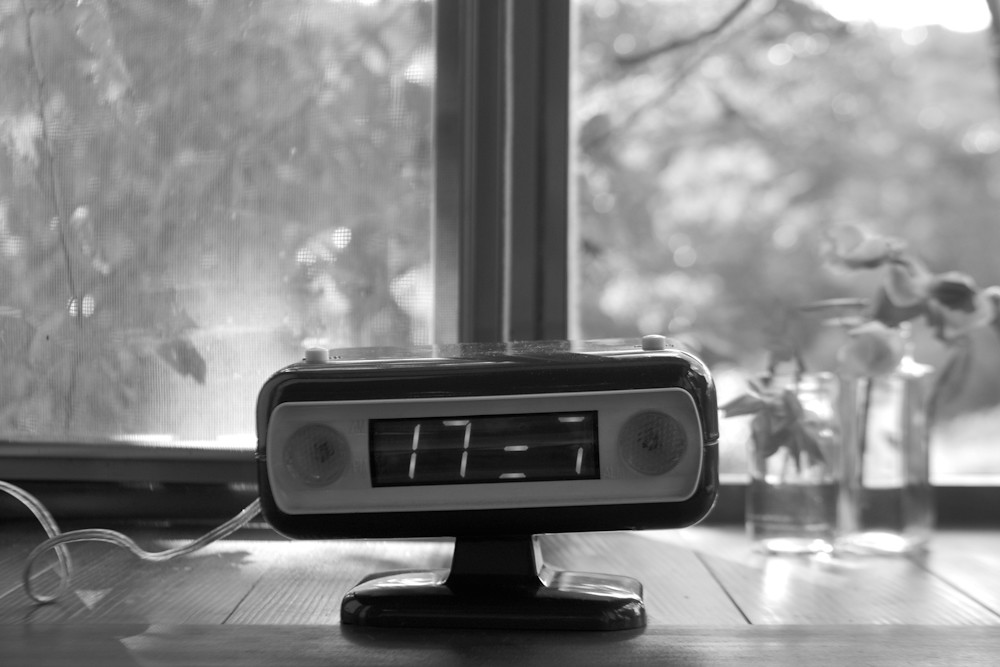A black and white photograph captures an oblong desk clock perched on a sleek black stand. The clock features a white face with a digital display that curiously reads "17 = 7," likely due to some malfunctioning segments of the display. On either side of the digital display are various buttons, and additional buttons can be seen on the top, one on the left and one on the right. The clock is positioned on a wooden window sill, adding a touch of rustic charm to the scene.